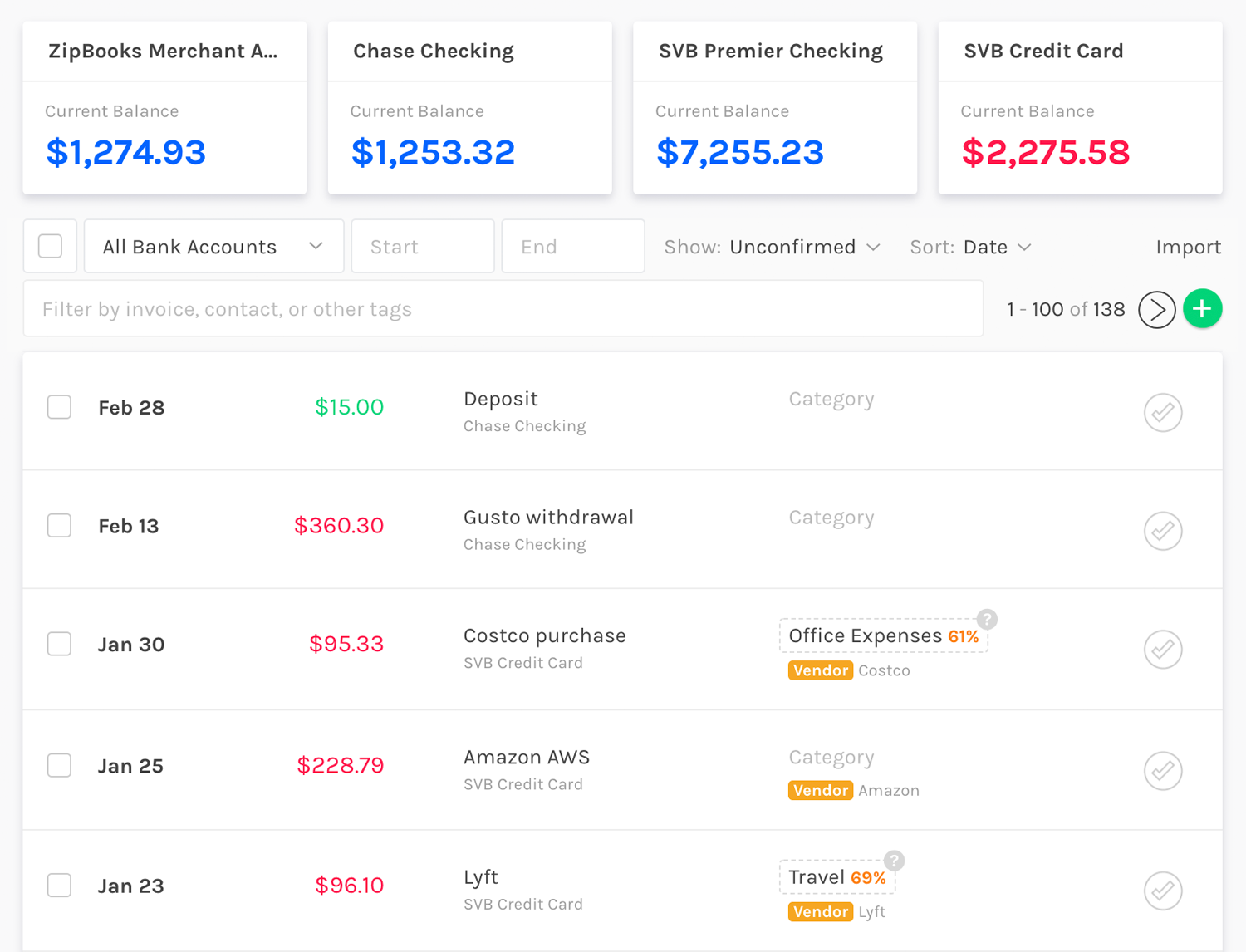The image features a financial dashboard displaying various sections with detailed account information. At the top, there is an account labeled "ZipBooks Merchant" showing a current balance of $1,274.93. The following section is "Case Checking," which has a balance of $1,253.32. Another section, "SVB Premier Checking," lists a balance of $7,255.23. Lastly, the "SVB Credit Card" section shows a balance of $2,275.58.

Below these accounts, a series of filters are available, including options to view "All Bank Accounts" and to set a "Start" and "End Date." There is a "Show" button, an "Unconfirmed" filter, and a "Sort by Date" feature.

Underneath these filters, a list of financial transactions is displayed with dates and details:
1. **February 28th**: A green deposit of $15 into the "Case Checking" account.
2. **February 13th**: A red withdrawal of $360.30 for "Gusto," categorized under "Case Checking."
3. **January 30th**: A red charge of $95.33 for a "Costco Purchase" on the "SVB Credit Card," categorized under office expenses (61%), and the vendor is listed as Costco.
4. **January 25th**: A red charge of $228.79 for "Amazon AWS" on the "SVB Credit Card," with Amazon as the vendor.
5. **January 23rd**: A red charge of $96.10 for "Lyft," categorized under travel (69%), with Lyft as the vendor, on the "SVB Credit Card."